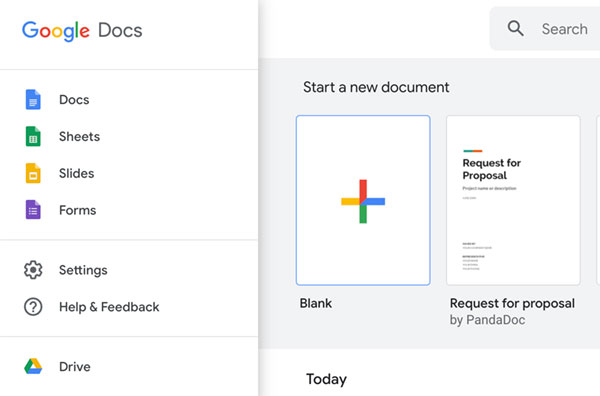The image shows a Google Docs page, showcasing various features and options available to the user. In the upper left corner, the "Google Docs" heading is displayed with "Google" in its iconic multicolored letters, while "Docs" is in dark gray. The interface is split into two sections. On the left side, a vertical menu provides access to different Google Workspace tools from top to bottom: Docs, Sheets, Slides, Forms, Settings, Help, and Feedback. At the bottom of this menu, there is a link to access Google Drive.

On the right side, in the upper right corner, there is a search box designed for navigating through the user's Google Docs. Below this search bar, an option to "Start a New Document" is available, depicted as an 8.5 by 11-inch sheet of paper with a plus sign in the middle, colored in Google's signature colors. Next to this, there is an already opened document titled "Request for Proposal," authored by a user named PandaDoc, which can be accessed directly from this menu.